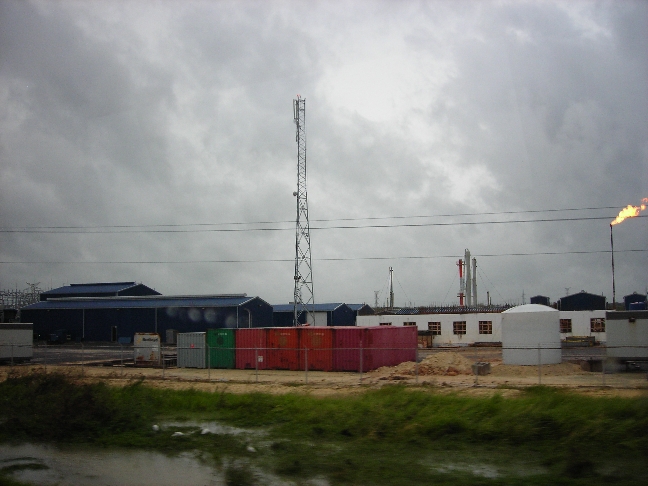The image captures a moody outdoor scene dominated by a vast, overcast sky that spans about two-thirds of the frame, casting a grey hue over the entire landscape despite it being daytime. In the foreground, vivid green grass can be seen, appearing waterlogged and glistening slightly, possibly from recent rain. Moving further back, there's a strip of sandy terrain leading to a cluster of metal cabins or storage units. These structures are predominantly painted red, although to the left, a couple of them stand out with green and grey exteriors. Further in the background, a blue-roofed structure can be observed, partially obscured by the cabins. Rising centrally from within the scene is a tall metallic frame, intricately laced with long telephone wires stretched taut across the cloudy sky, adding a layer of industrial complexity to the otherwise serene, yet somber, landscape.